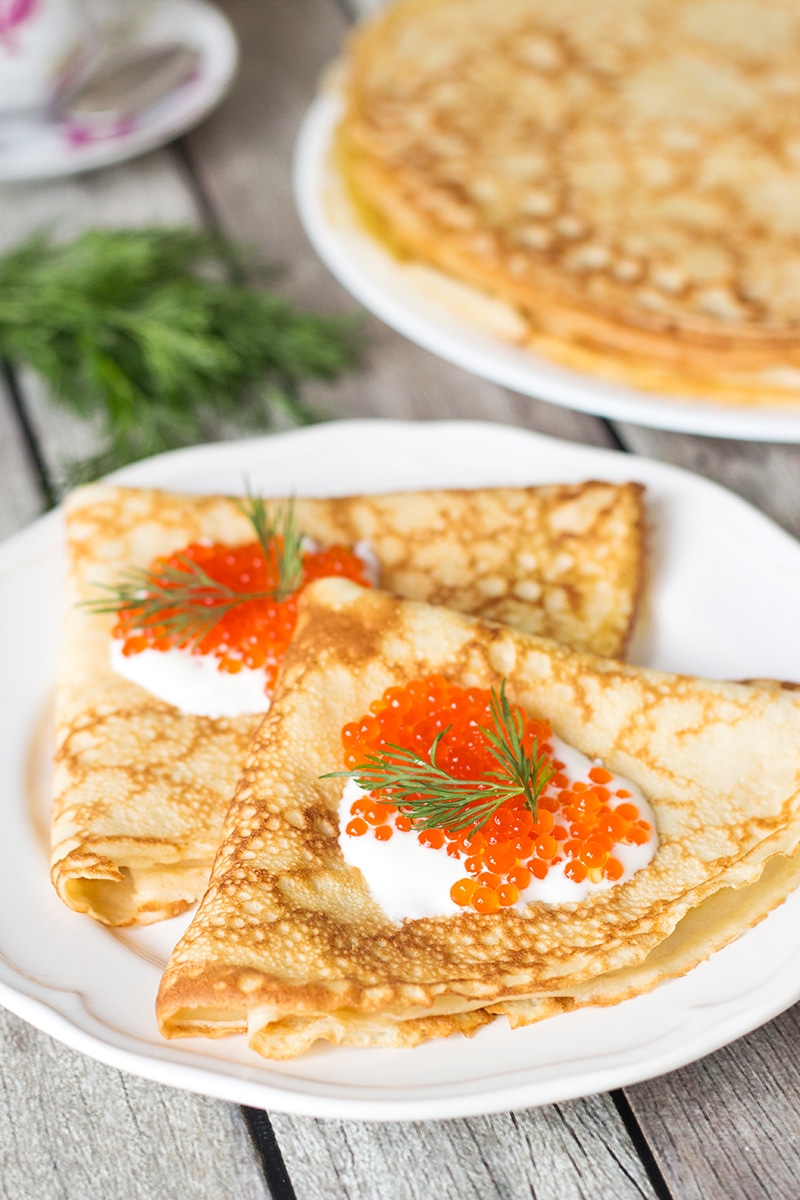This is an exquisitely presented photograph of food featuring two white plates resting on a weathered gray wooden table. The focus is on two folded crepes in the foreground, each topped with a dollop of white sour cream and sprinkled generously with bright red caviar. Each crepe is garnished with a sprig of green dill, adding a touch of freshness. The crepes are artfully layered, their golden-brown surfaces hinting at perfect cooking. In the background, slightly blurred, are additional flat crepes on another white plate, accompanied by a small bunch of fresh dill to the left. The table's textured, gray surface enhances the rustic, inviting appeal of the scene, evoking a cozy, elegant presentation ideal for a delightful meal.